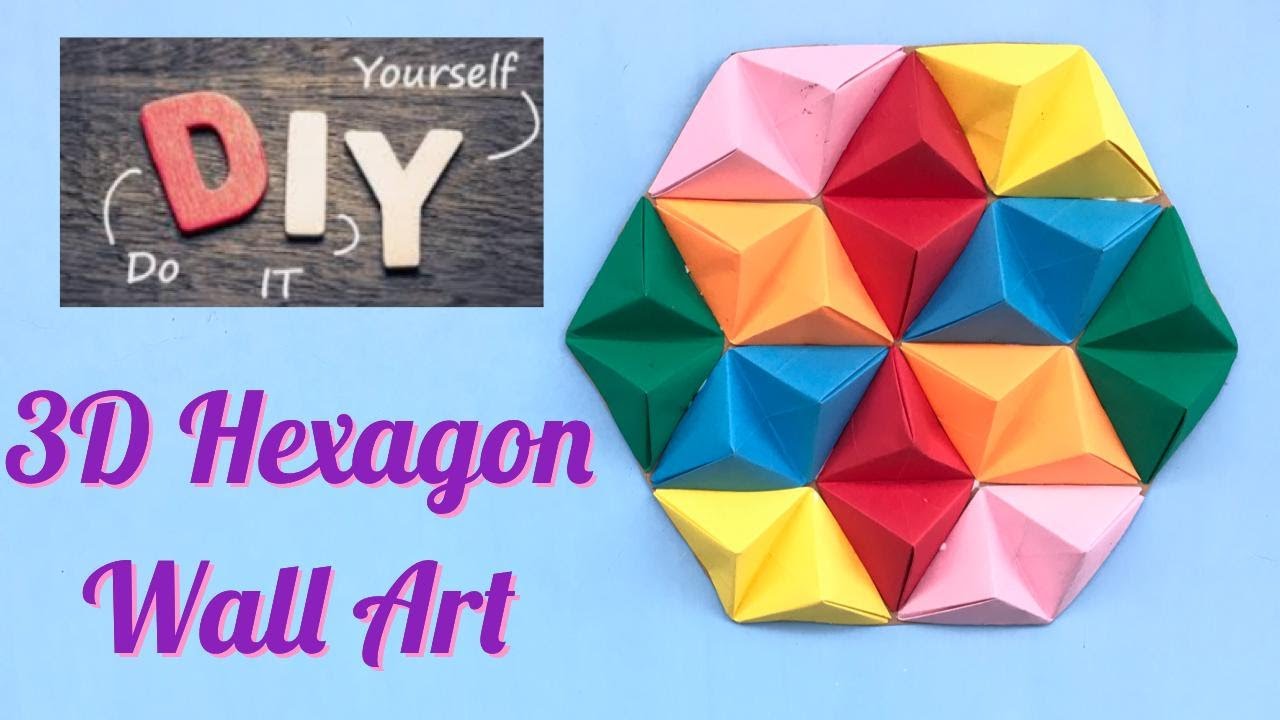This is an advertisement for DIY 3D Hexagon Wall Art, presented in a rectangular, landscape format. In the top left corner, the acronym "DIY" is displayed with the "D" in red and the "I" and "Y" in a whitish-yellow color. The letters are stylized with a script that extends lines from the "D" to "Do," under the "I," and above "yourself," against a dark wood background. Directly beneath, in purple type, it reads "3D Hexagon Wall Art." The right side of the image features a hexagonal wall art piece composed of variously colored origami-like paper pieces—red, yellow, light pink, blue, green, and orange—arranged to form a star shape at the center, all set against a light blue background.